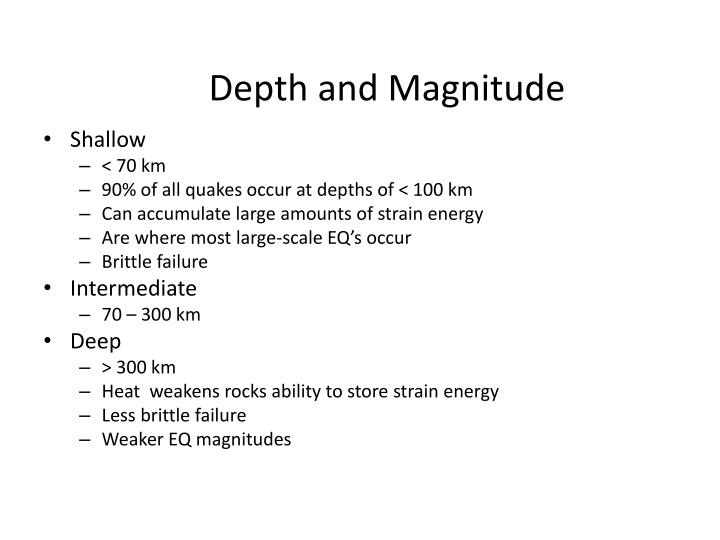The image features a black text presentation on a white background titled "Depth and Magnitude" in large font. Beneath the title, there are three bulleted categories: Shallow, Intermediate, and Deep, each with associated sub-bullets providing further detail. 

- Shallow: 
  - Defined as less than 70 kilometers deep.
  - 90% of all earthquakes occur at depths less than 100 kilometers.
  - Can accumulate large amounts of strain energy.
  - Where most large-scale earthquakes occur.
  - Characterized by brutal failure.
- Intermediate:
  - Ranges between 70 to 300 kilometers in depth.
- Deep:
  - Depths greater than 300 kilometers.
  - Heat weakens the rocks' ability to store strain energy.
  - Less brutal failure.
  - Weaker earthquake magnitudes.

The text offers detailed information likely related to seismology, suggesting its use in a science class or professional presentation. The layout resembles a slide from a lecture or educational presentation addressing the characteristics and impacts of earthquakes at varying depths.